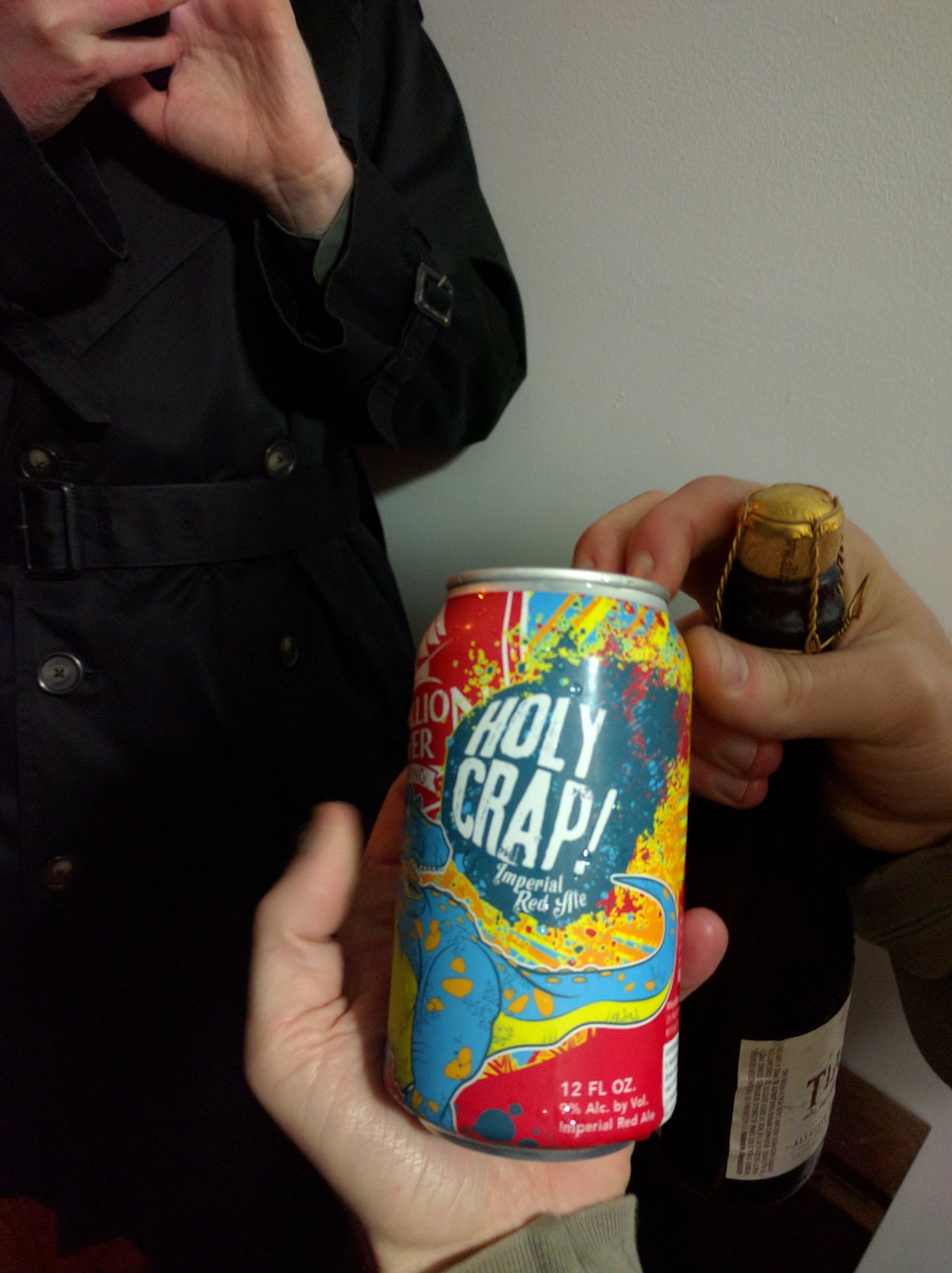A dynamic photograph captures a moment of lively celebration. In the upper left corner, a person facing the camera dons a long-sleeved black jacket, their hands raised in front, concealing their face. In the bottom right corner, a second pair of hands is engaged in a jubilant toast. The left hand clutches a vividly colorful can labeled "Holy Crap! Imperial Red Ale," while the right hand holds a dark bottle of champagne or sparkling wine, adorned with a gold foil top and a securing cage. The champagne bottle's white label, partially obscured, reveals only a prominent letter 'B,' hinting at the mysterious brand. The contrast between the vivid can and the elegant champagne bottle underscores the diversity of the celebration.